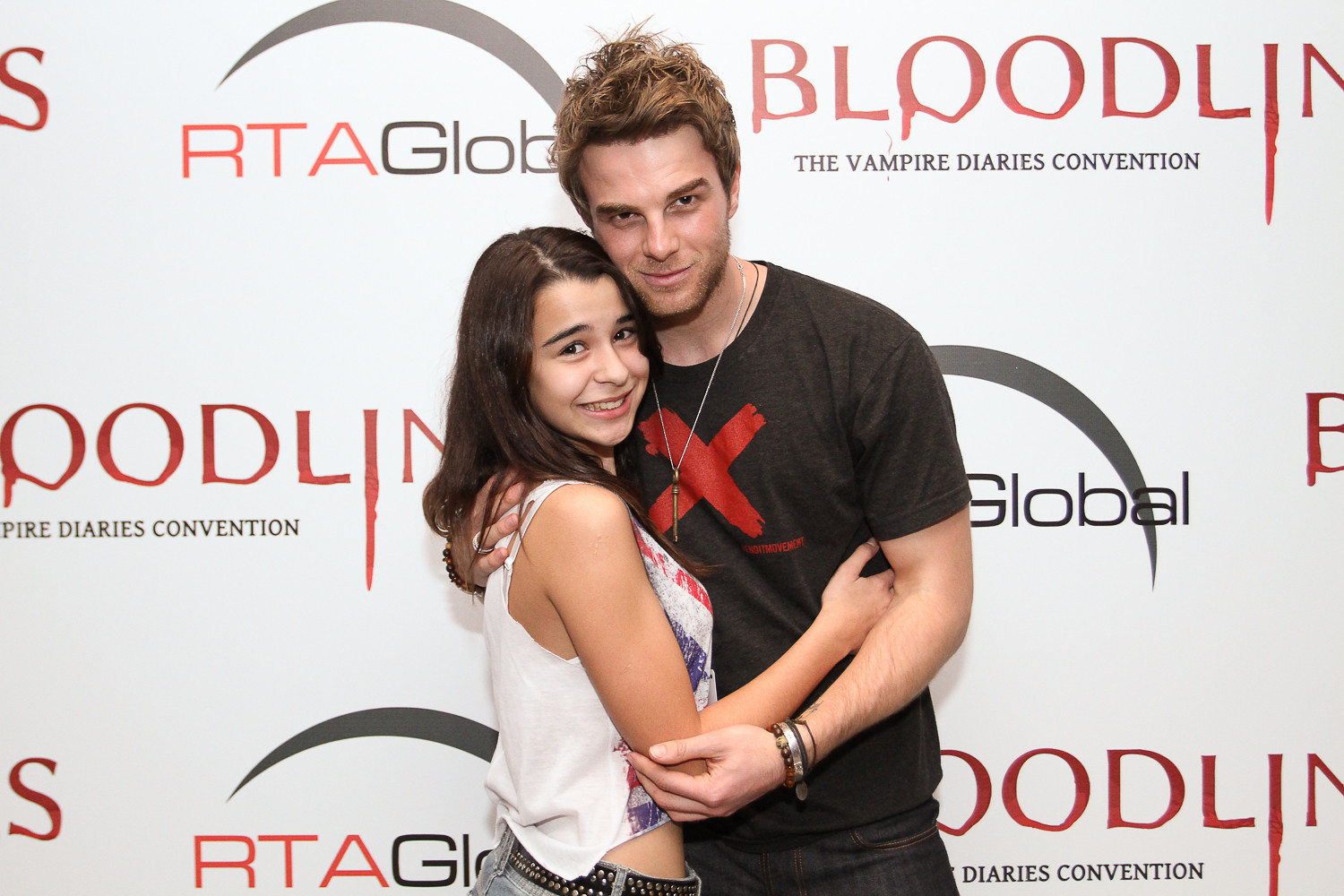In this photograph, a young girl and a slightly older guy are standing close together, with their arms wrapped around each other, smiling warmly at the camera. The girl, positioned on the left, has shoulder-length dark hair and is dressed in a white tank top that features a red and blue graphic print on the front, paired with jeans and a black studded belt. She appears to be in her late teens or early adulthood. The guy, to the right, is a white male with tips of light brown in his dark hair and sports a 5 o'clock shadow beard and mustache. He is wearing a black t-shirt with a red X on the front, dark denim jeans, and a necklace featuring a key. They are posing against a white wall adorned with the text "RTA Global, Bloodline, The Vampire Diaries Convention." The overall background and their attire suggest a casual and upbeat atmosphere, possibly indicating that the guy is a public figure at an event and the girl is excited to meet him.